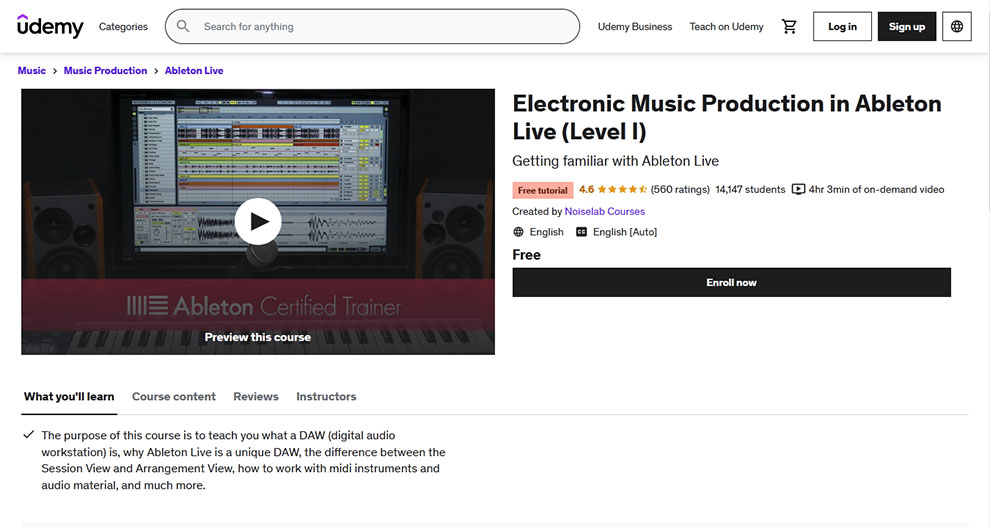This is a detailed caption for the given image description:

---

Screenshot of the Udemy website showcasing an online course titled "Electronic Music Production in Ableton Live Level 1." The page features a prominent "Enroll Now" button, indicating that users can purchase and start the course. The course is taught by an Ableton Certified Trainer and offers a brief preview video displaying an equalizer interface, demonstrating how to layer and manipulate various tracks to create music. The course description outlines key learning objectives, including understanding what a Digital Audio Workstation (DAW) is, exploring the unique features of Ableton Live, distinguishing between Session View and Arrangement View, and mastering the use of MIDI instruments and other music production materials.